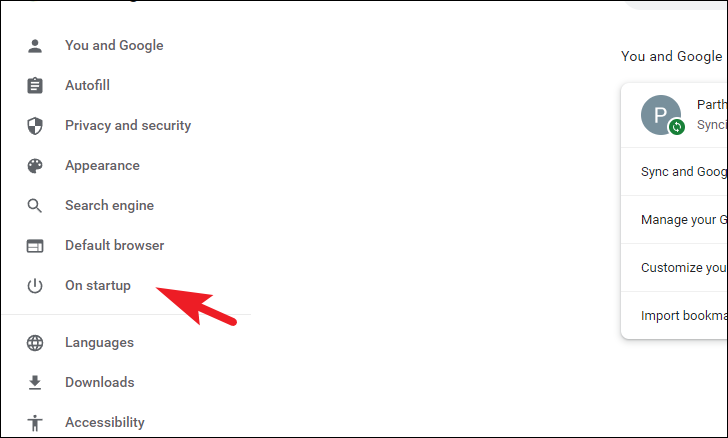This image is a detailed screenshot of a computer's browser settings page, featuring a white background. On the left side, the view is slightly zoomed in, displaying a vertical, gray, mixed-case menu. At the top of the menu is a silhouette icon of a person’s head and shoulders, labeled "You and Google." Below it are several menu items: "Autofill," "Privacy and Security," "Appearance," "Search Engine," "Default Browser," and "On Startup," which is highlighted by a large red arrow pointing at it. Further down, the menu continues with "Languages," "Downloads," and "Accessibility."

To the right of this menu, partially visible, is a section titled "You and Google." This section features a blue circle with a white letter "P," likely representing the user’s avatar. The text here includes options for "Sync Google," "Manage Your Account," "Customize Your Account," and "Import Bookmarks." The overall scene suggests the user is engaged in browsing or managing their browser's settings, specifically focusing on startup configurations.